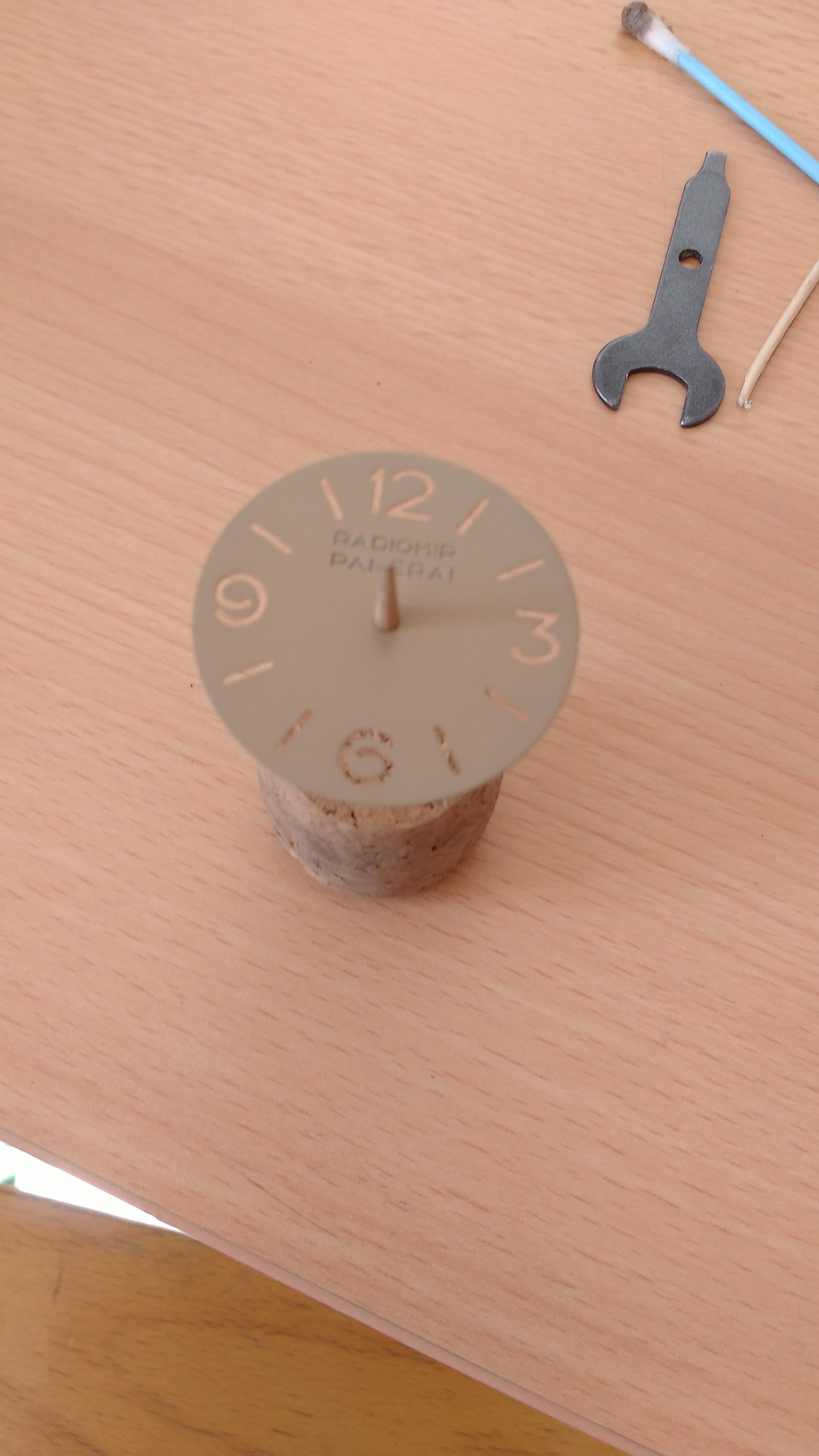On a light wooden countertop, a small gray wrench with a hole in the middle sits at the top right corner. To its left, there is a white q-tip with a darkened tip. Positioned at the bottom right is a white toothpick against the wooden surface. Centrally, there is an object resembling a radio with a circular face, featuring dials and indicators. The numbers 12, 3, 6, and 9 are marked at the top, right, bottom, and left positions respectively, with two dash markers between each set of these cardinal numbers. The dial is predominantly gray, and there's a stone-like structure beneath it. The countertop itself is light wood, transitioning to a brown hue at the bottom of the image.